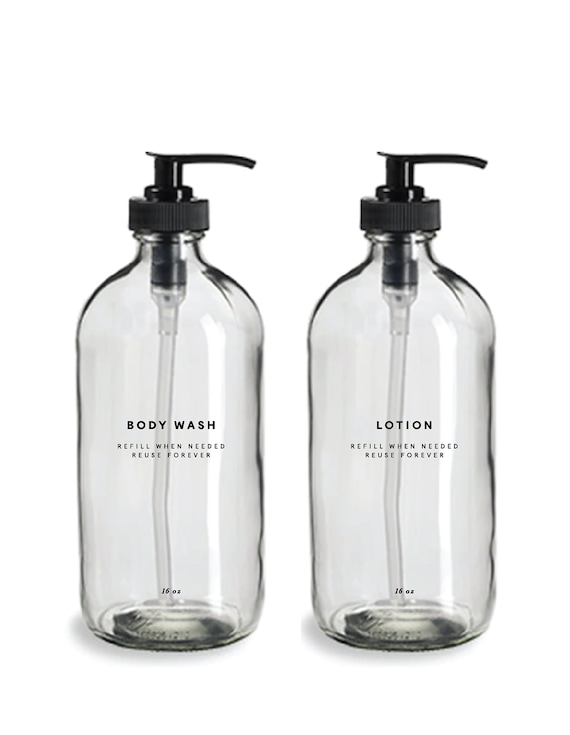The photograph depicts two identically sized, clear glass pump bottles, each with a volume of 16 ounces. The left bottle is labeled "body wash," and the right one is labeled "lotion." Both labels bear the environmentally conscious message, "refill when needed, reuse forever." Each bottle is equipped with a black plastic pump mechanism, with a clear plastic tube extending down into the bottle. A maker's mark or label indicating "16 ounces" is visible at the bottom of both bottles. The bottles stand upright against a pure white background, suggesting that the image is suitable for a catalog or a product listing on a website. The dimensions appear to be a few inches in diameter and approximately five to six inches in height.